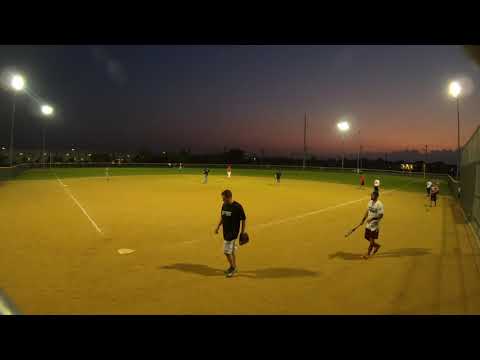This detailed nighttime photograph captures a baseball game in progress on a sports field illuminated by stadium lights against a multi-colored dark sky, ranging from reddish to purple hues. The infield is noticeably sandy or tan-colored, marked by white baselines for first and third. The outfield contrasts with its green grass. Prominently in the foreground, two players can be seen: one in a black short-sleeve shirt with white shorts and sneakers, wearing a glove, and the other in a white shirt with dark or brownish shorts, holding a bat and walking toward the first player. Shadows of these players stretch across the field. Scattered across the field are additional players, including several in the infield and at least one in the outfield, though details become less distinct with distance. The field is framed by horizontal black strips above and below, likely part of the photograph's format.